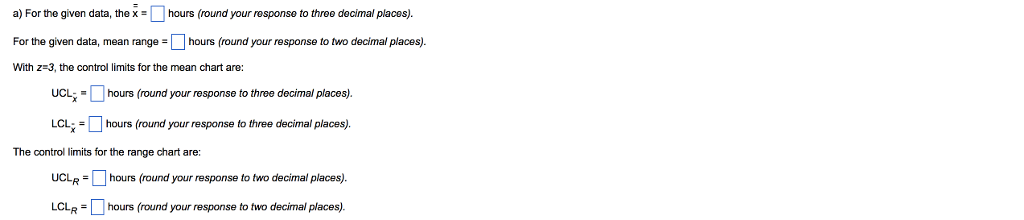**Detailed Caption:**

The image features a sample test on a white background, focusing on control chart calculations. The test offers several sections that require specific inputs:

1. **Given Data:**
   - Variable A is provided.
   - Variable X is to be calculated and entered in a box, with responses rounded to three decimal places.

2. **Mean Range Calculations:**
   - The mean range (denoted as R) needs to be entered in a box, with values rounded to two decimal places.

3. **Mean Chart Control Limits:**
   - **Upper Control Limit (UCL):**
     - UCL for X requires a response entered in a designated box, rounded to three decimal places.
   - **Lower Control Limit (LCL):**
     - LCL for X also requires an entry in a box, rounded to three decimal places.

4. **Range Chart Control Limits:**
   - **Upper Control Limit (UCL) for Range:**
     - UCL for R needs to be entered in a blue box, with values rounded to two decimal places.
   - **Lower Control Limit (LCL) for Range:**
     - LCL for R requires a response in a box, also rounded to two decimal places.

Each section clearly indicates the unit of measure as hours and specifies the required decimal precision for the responses.